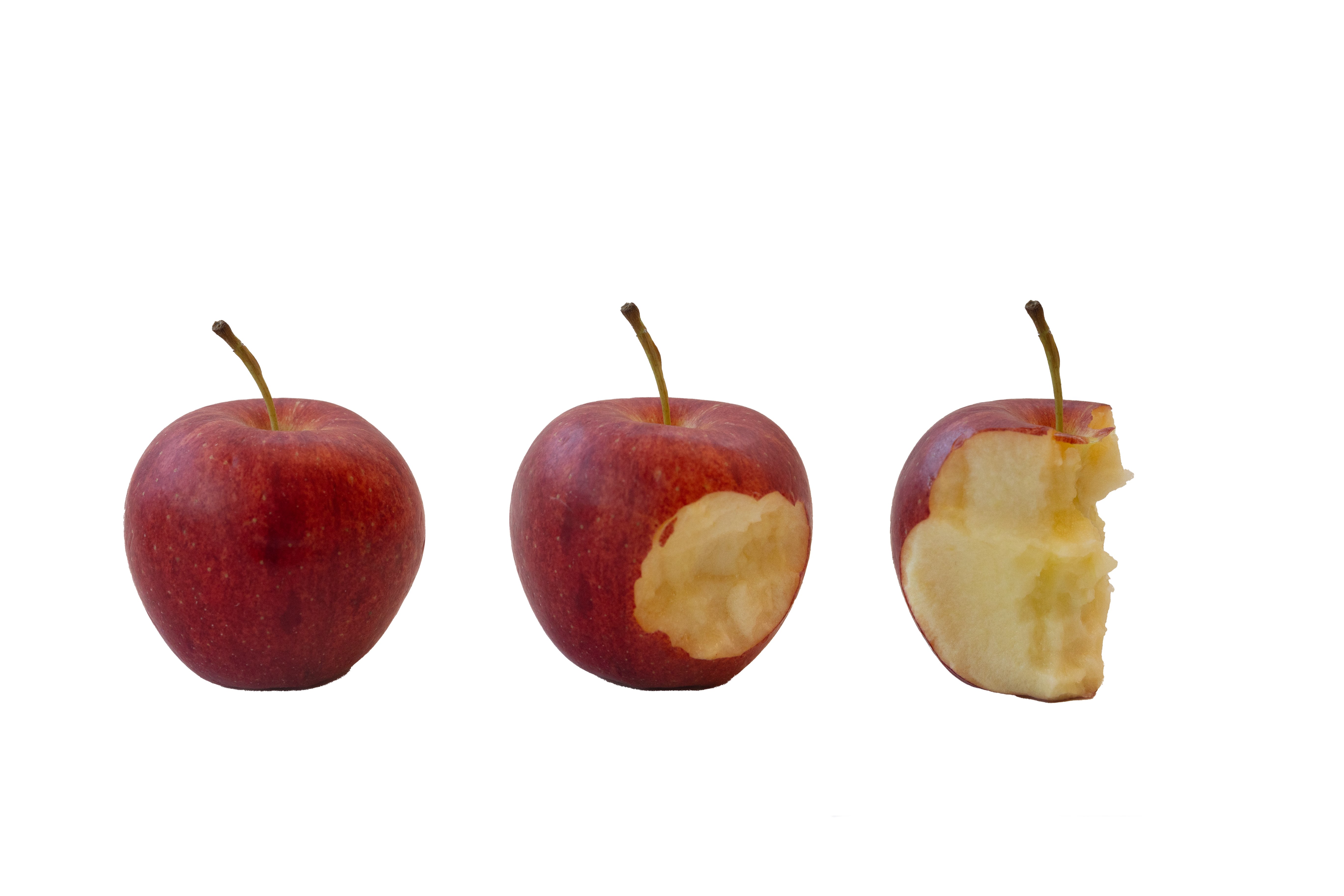This image, set against a simple white background, depicts three stages of a red apple being eaten, arranged horizontally from left to right. The first apple on the left is whole, characterized by its vibrant red skin with various splotches and minor defects, and a slightly curved green and brown stem. The middle apple shows a significant progression, with a large bite taken out, exposing the white interior and teeth marks on the right side. The third apple, on the far right, is nearly consumed, with three-quarters of it eaten away, leaving only a sliver of the red outer skin and the core visible, while the stem remains intact. The sequence illustrates the transformation of the apple as it’s being eaten, all set against a minimalist background.